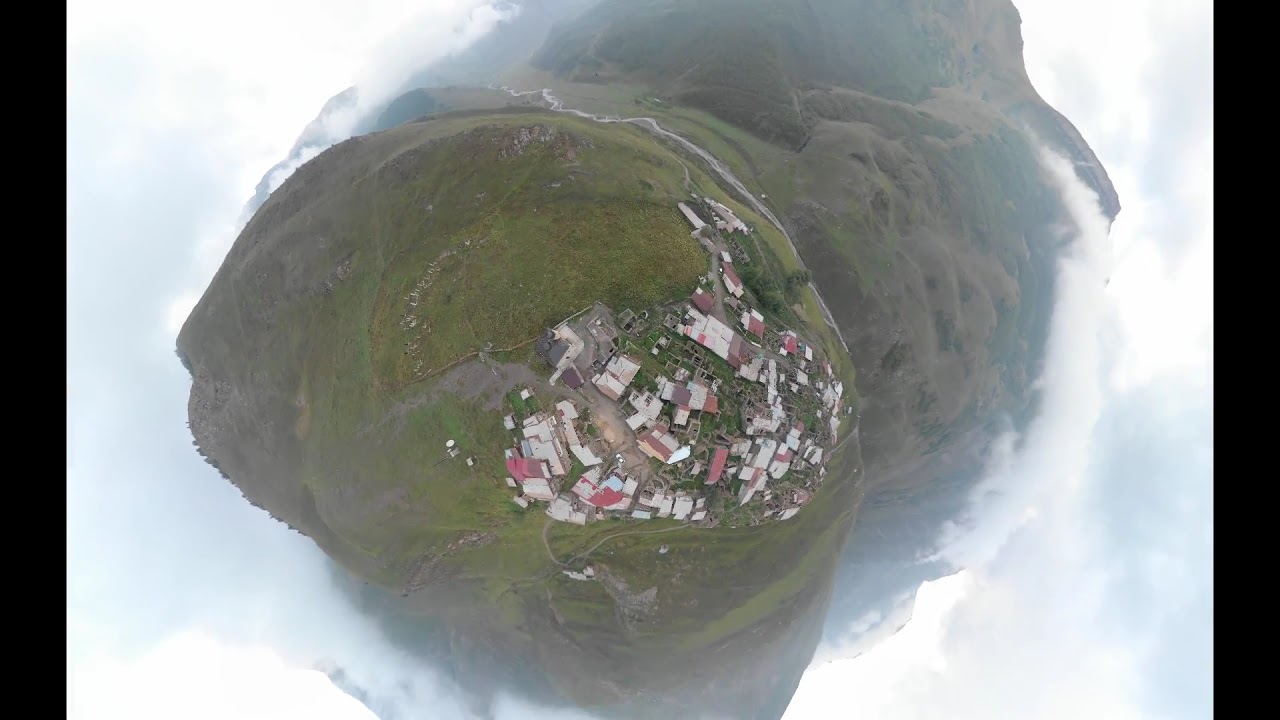This image captures a unique aerial view, looking straight down onto the top of a mountain, distorted by an unusual lens that makes everything appear very curved, almost as if looking at a Tootsie Roll or a long piece of bread. The mountain itself is lush and green, with a closely-packed city perched precariously near its edge. The city is characterized by buildings with red, white, and brown roofs, giving a vivid yet compact appearance. Below the city, the mountain's rounded contours are visible, some sections densely forested with trees, while others are more barren, covered in green grass. The entire mountain is encircled by a mix of white clouds and patches of blue sky, contributing to the serene yet surreal visual. The image further encompasses thick black lines running horizontally down either side, adding to the distorted appearance. A winding road snakes through the area, dotted with white, red, and tan houses, and a brown dirt pathway. Despite the slightly confusing perspective, possibly taken from a drone or with a specialized lens, the photo provides a fascinating glimpse of a city seemingly melding into its mountainous surroundings amidst patches of foggy white and blue sky.